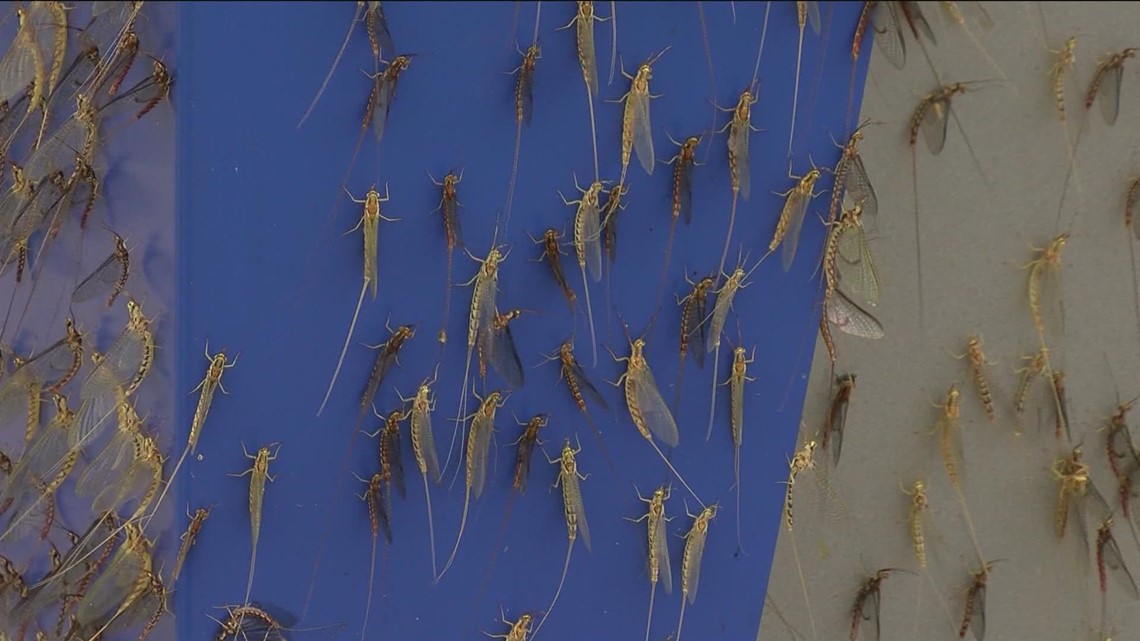This image captures a multitude of fascinating insects on a vertical, bluish-gray striped surface. These insects, possibly dragonflies or grasshoppers, have long bodies, thin and elongated tails, and transparent wings that match the length of their bodies. Their prominent antennas and legs contribute to their intricate appearance. The insects vary in color from light beige to a darker brown, scattered throughout the blue central stripe flanked by gray and dull blue sections. All the insects are facing upwards, seemingly climbing up the wall in a scattered formation, creating an intriguing visual display.